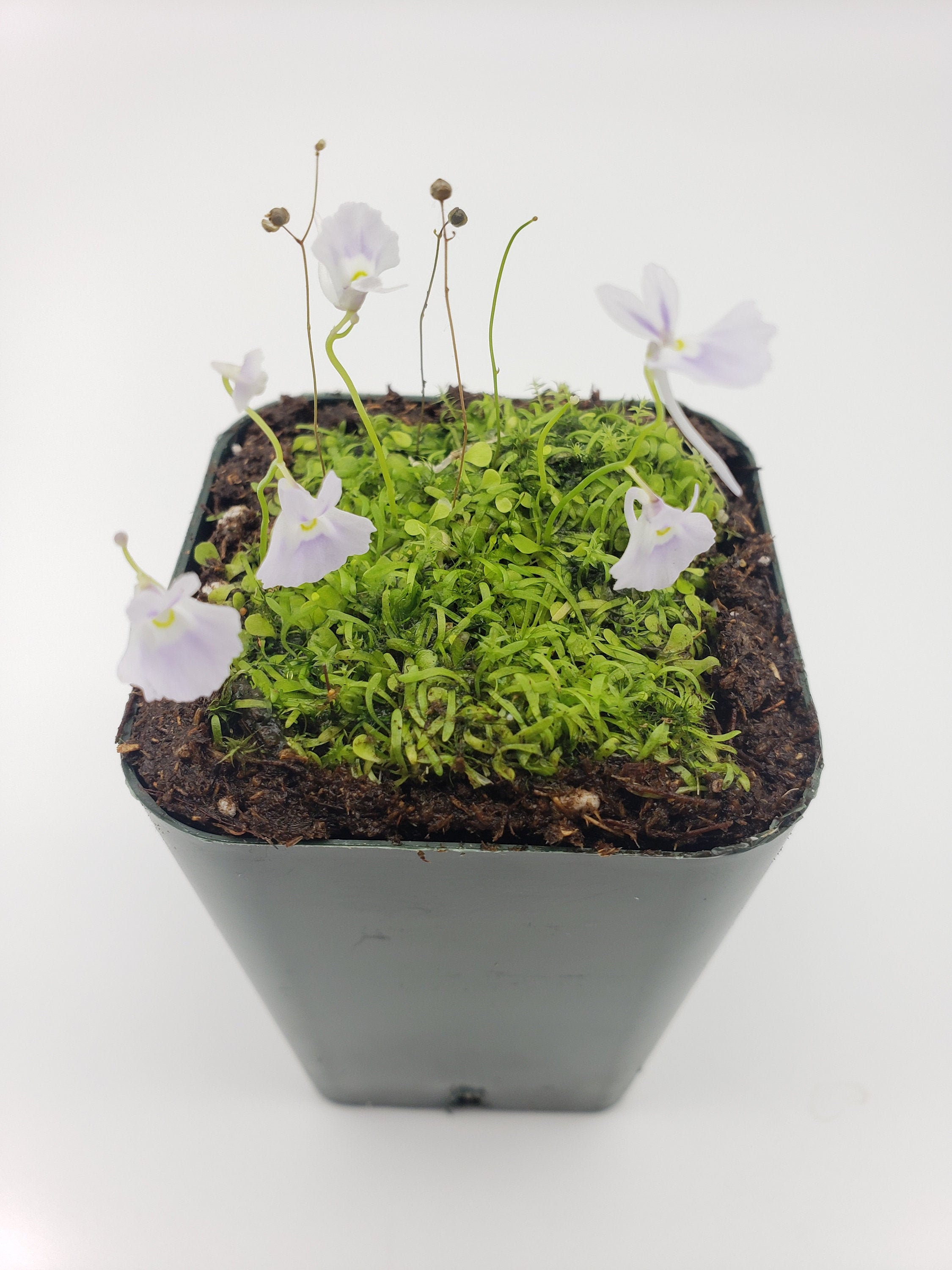A potted plant with a white base sits centrally against a stark white background. The planter is a tall, rectangular gray bin, viewed slightly from above at a diagonal, causing it to appear larger at the top and narrower towards the bottom. The edges of the bin are filled with dark brown soil, resembling a garden border, and the center contains small, curly green grass. Among the grass, there are several thin twigs with unopened bulbs, and six white flowers in various stages of bloom, with some petals drooping downwards. The detailed arrangement makes the plant look meticulously nurtured in a mini-garden setting.